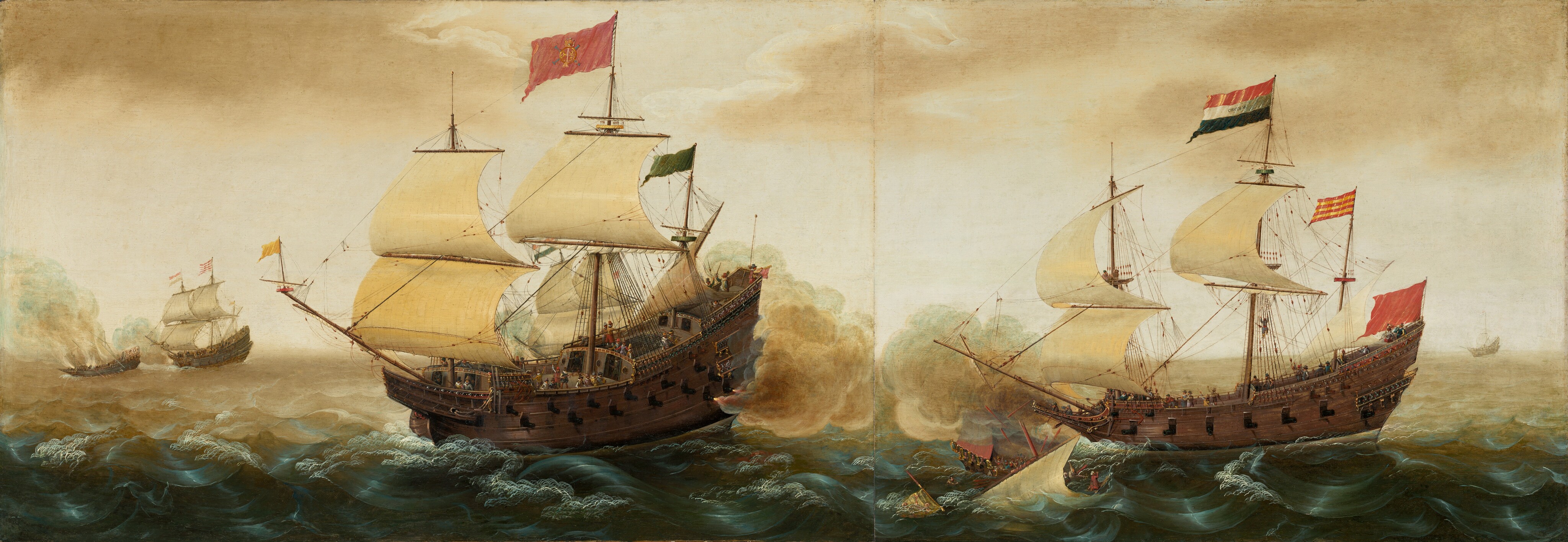The painting illustrates a dramatic naval battle set in the turbulent seas of the 17th century. In the foreground, two majestic ships with towering wooden masts and billowing white sails engage in fierce combat, their cannons firing at one another. The vessel on the left, bearing a red flag, exchanges fiery blasts with the ship on the right, which hoists a striped flag of red, white, and blue. Between them, the remains of a shipwreck add to the scene's intensity, while the raging blue waves crash around them. In the background, additional ships, some enveloped in flames and smoke, struggle amidst the chaos. The sky above is a tumultuous blend of yellow, beige, and smoky brown, adding to the dramatic atmosphere of this historic maritime clash.